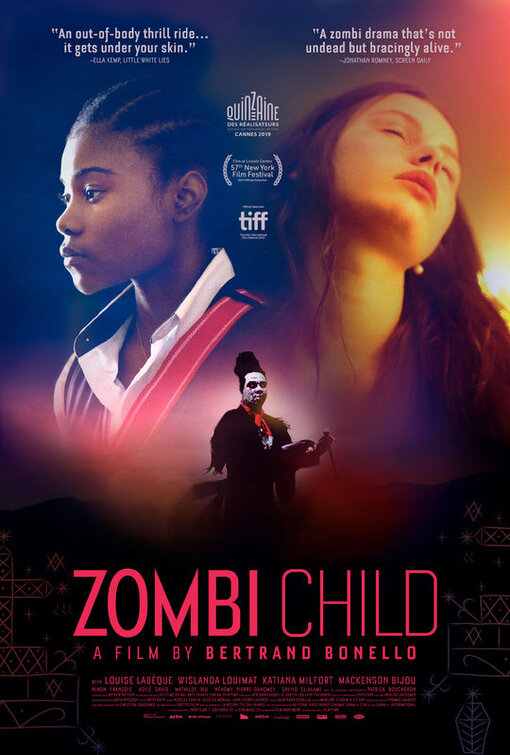The poster showcases a dramatic advertisement for the movie "ZOMBIE CHILD," set against a dark background. At the top, white text reviews praise the film, calling it "an out-of-body thrill ride" and "a zombie drama that's not undead but bracingly alive." Central to the poster are three characters: on the left, a young woman with dark skin and braided hair gazes solemnly to the left; on the right, another woman with light skin, brown hair, and closed eyes tilts her head as if in deep thought. Dominating the center is a menacing figure with a white painted face, a tall black hat, and black attire, possibly holding a knife. This character's eerie presence adds to the film's chilling allure. Below this striking imagery, in bold pink letters, is the movie title "ZOMBIE CHILD," followed by "A FILM BY BERTRAND BONELLO" and detailed credits for the producers, actors, and directors. The overall aesthetic of the poster is dark and immersive, setting a foreboding tone fitting for a horror film.